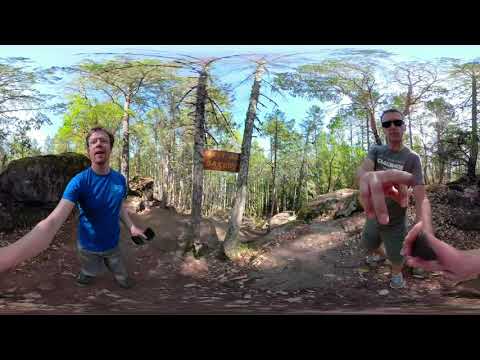The image, taken with a GoPro 360 lens, features two white men in a forest setting, creating a slightly distorted effect with morphed edges and black horizontal borders at the top and bottom. The man on the left, in a blue t-shirt and gray pants, has short brown hair and stretches his arms outward, holding the camera in his right hand and an unidentified object in his left. The man on the right, slightly darker-skinned, wears black sunglasses, a light brown shirt, and olive green shorts. He gestures towards the camera with his pointing finger. The ground is strewn with dirt, scattered rocks, and dry brown leaves. Two central trees bear a wooden camp sign, while the background reveals a mixture of barren and sparsely green trees under a bright blue sky with scattered clouds, depicting a daylight scene.